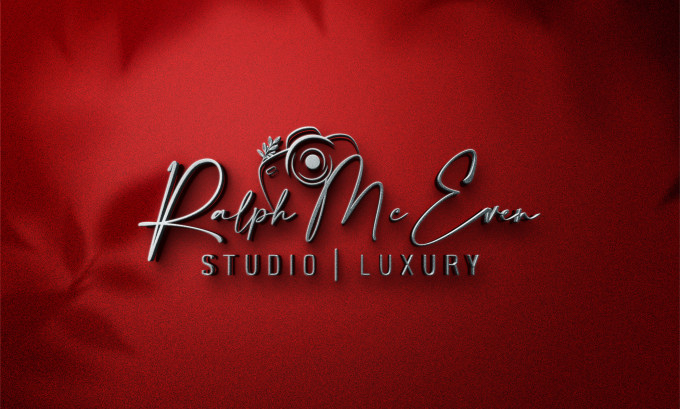The image showcases a distinctive graphic design logo against a velvety red background that darkens towards the corners. At the center, the name "Ralph McEwen" is elegantly written in cursive, with a unique detail resembling a small camera lens or circle located between the 'P' and 'M'. Extending from this circle is a leaf-like design that adds a touch of nature to the sophisticated layout. Directly beneath the name, the phrase "STUDIO | LUXURY" is inscribed in grey, all-caps text, separated by a vertical line. The background is adorned with subtle shadows of leaves: the top left corner features elongated, creeping leaves, while the bottom left corner includes a twig with protruding leaves. Overall, the intricate detailing and rich colors convey a sense of luxury and elegance.